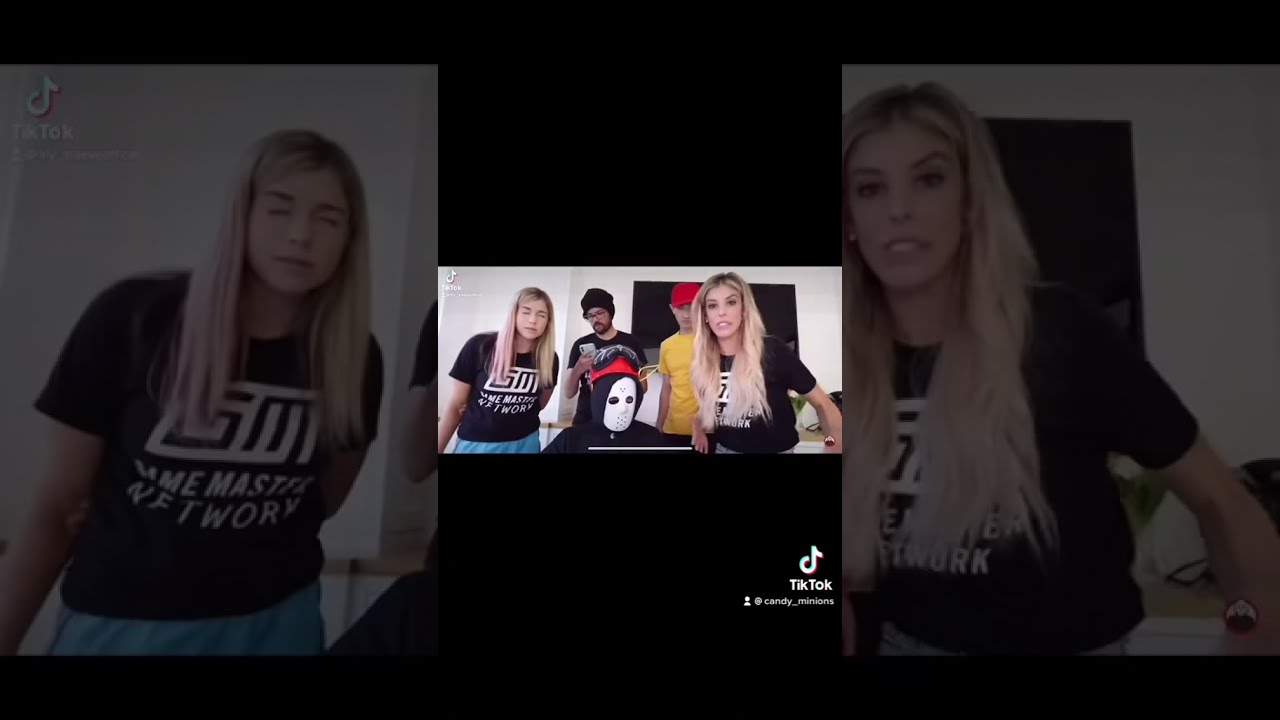A TikTok image, likely captured with a phone camera in landscape mode, showcases a group of five individuals in what appears to be a living room setting. The main focus is a man sitting in the center, donning a white hockey mask with a black hood pulled over his head and a red crown on top. Flanking him are two similar-looking blonde girls—one with straight hair and the other with wavy hair—both wearing identical black and white shirts with the word "work" visible on them. You can only see them from the hip up. In the background, there is a guy in a black ensemble—a black shirt, a black beanie, black glasses, and sporting a handlebar mustache with a beard, who appears to be looking at his white cell phone. Another man, distinguishable by his yellow shirt and red hat, is also visible. The backdrop features a white wall with what seems to be a TV mounted on it. The entire setup is framed by a darkened, zoomed-in version of the same image, adding a dramatic filter over the background. The bottom right corner displays a TikTok symbol alongside the handle "at candy_minions."